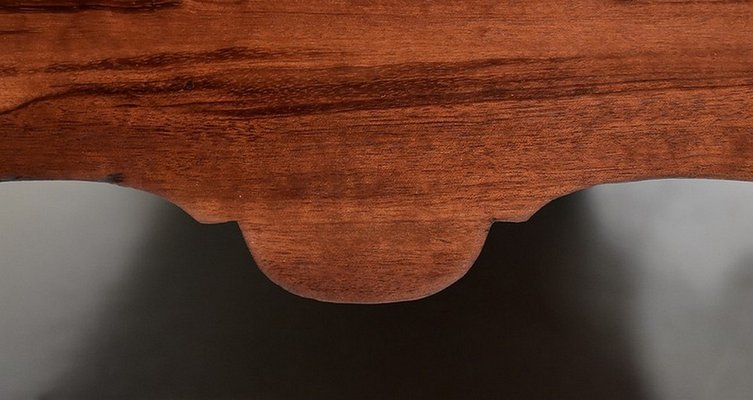This image presents a close-up view of a wooden piece of furniture against a dark, reflective background. The wood, possibly oak with rust-colored hues and darker striations, features an intricate design. The central detail includes a horizontal segment from which two arches gracefully curve downward, flanking a circular motif with additional arches extending below. The reflected light on the dark background adds contrast, enhancing the piece's sheen. Though the specific object remains undetermined due to the close crop, it is speculated to be part of a decorative frame, potentially a headboard, the upper trim of a mirror, or the detailed underside of a piece of furniture such as a table or desk.